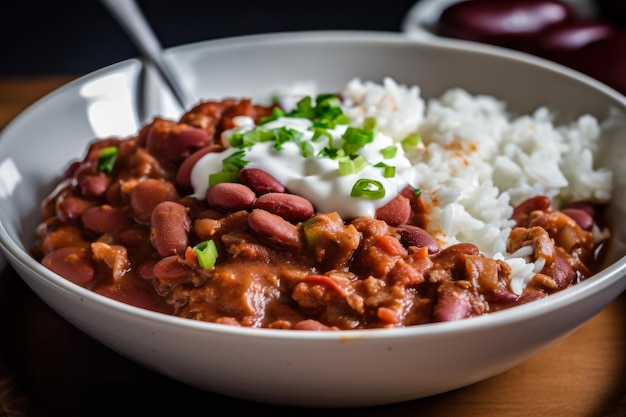The photograph captures a bowl-shaped, light gray ceramic plate with glossy, finished porcelain, sitting on a medium brown wooden table. This plate contains a hearty serving of white rice positioned toward the back right. On the opposite side, a generous portion of dark reddish-orange chili, rich with kidney beans and minced beef, is topped with a dollop of sour cream and garnished with chopped green onions. A gray spoon is tucked into the chili on the top left side. The image background features a blurry, dark red object in the top right corner, possibly a bowl of eggplants, further adding to the inviting, homely aesthetic of the setting.